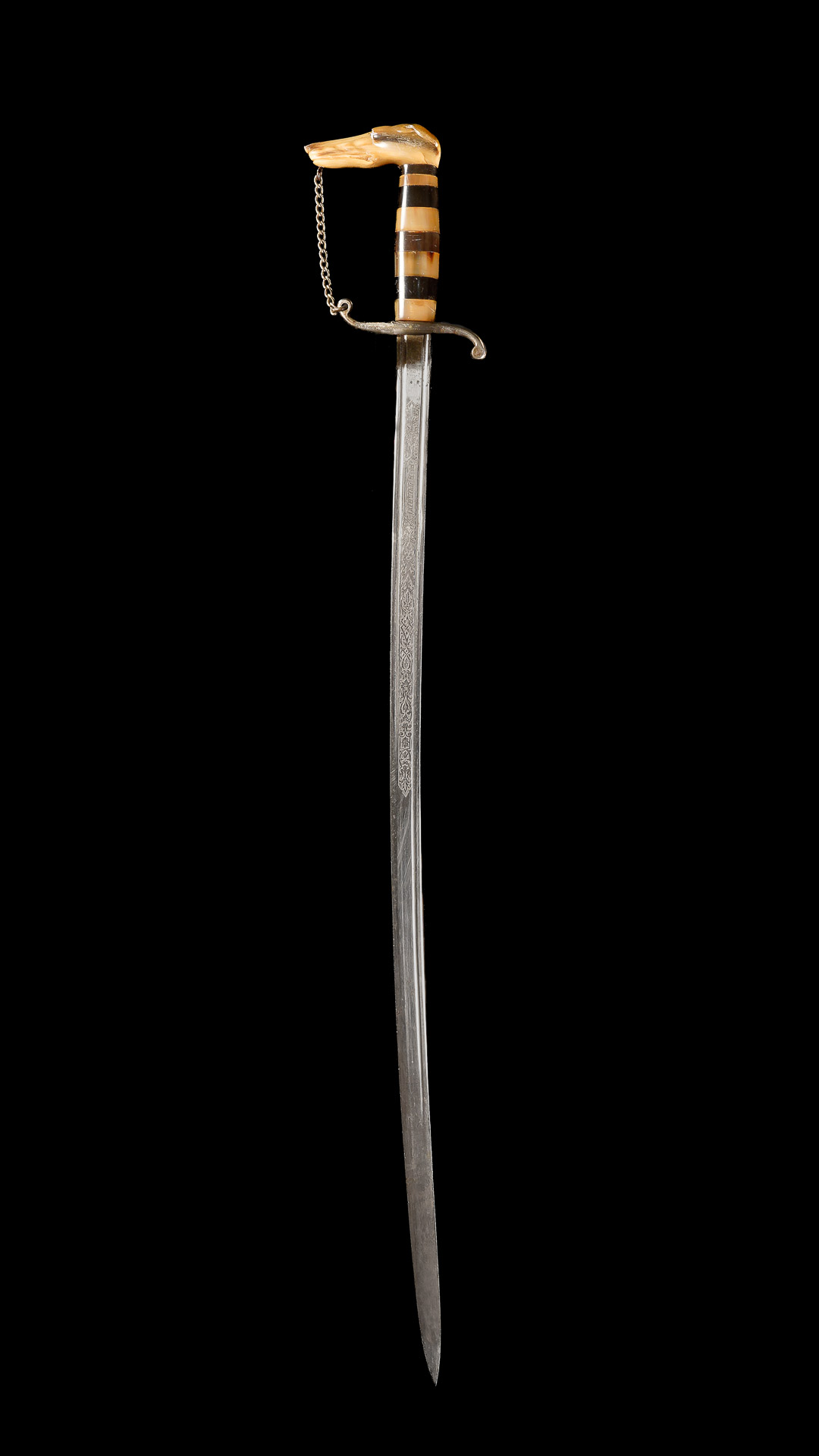This photograph showcases a finely-crafted, antique sword set against a stark, uninterrupted black background. Dominating the center of the image is the vertically-positioned sword, with the hilt at the top and the blade pointing downward. The sword features an intricately designed blade of silvery metal, adorned with elegant engravings on the upper half, though the resolution limits the visibility of finer details. The blade, measuring approximately 4 inches in length and 1/8 inch in width, appears slightly dulled and less reflective, suggesting its age and artifact status.

The hilt and handle are made of what appears to be natural, well-polished wood, showcasing a distinctive beige and brown striped pattern. The handle is accented with black rings, enhancing its aesthetic appeal. The hand guard, crafted from metal, extends horizontally and features unique, asymmetrical curves: it bends downward on the right side and upward on the left. A notable feature is a metal chain that springs from the hand guard and loops up to a subtle wooden extension at the top left of the handle, hinting at a secondary function, perhaps as a walking stick.

Overall, the composition and build suggest a robust design, evident in the detailed craftsmanship of both the blade and the handle, making it appear both a work of art and a potentially lethal weapon.